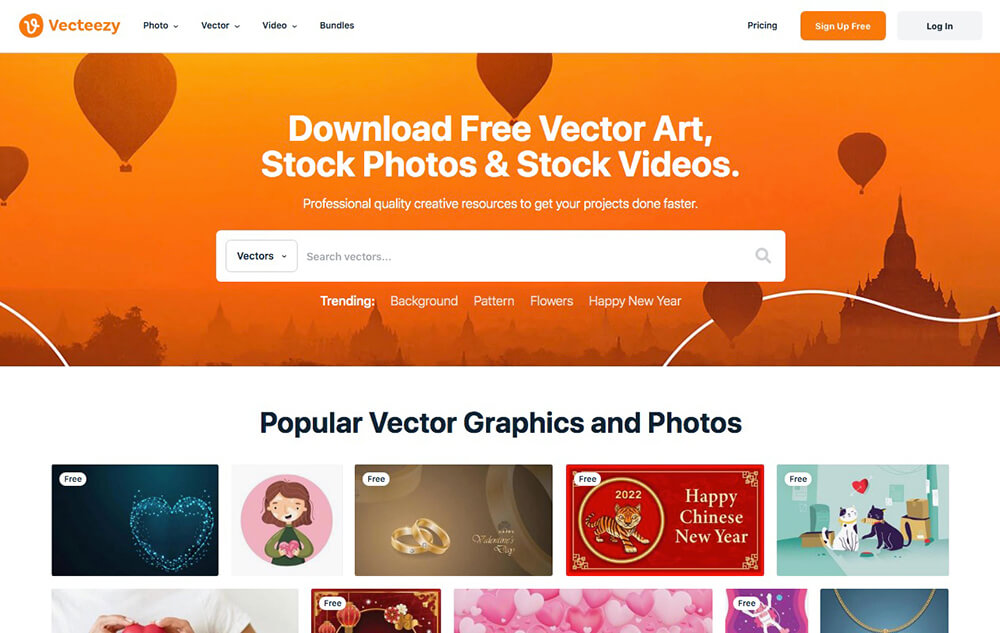This screenshot showcases a vibrant web interface featuring various graphical elements related to VectEasy. Situated in the top left corner, the VectEasy logo is prominently highlighted in orange. To the right of the logo appears the main navigation bar in a sleek white strip. This bar hosts several clickable options: "Photo," "Vector," "Video," and "Bundles" on the left side, while the right side is occupied by options for "Pricing," a distinct orange "Sign Up Free" button, and a gray "Log In" button.

Below this navigation strip, a striking orange banner spans the width of the page, featuring an artistic representation of balloons floating over what appears to be a cityscape. Centrally placed in white text on this banner is the inviting message, "Download Free Vector Art." Directly underneath, smaller text offers additional resources, including "Stock Photos" and "Stock Videos."

A white search bar is conveniently located beneath this banner, providing users with easy access to search functionality. Lastly, a series of categorized links are arrayed below the search bar, guiding users to popular sections such as "Trending," "Background," "Pattern," "Flowers," and "Happy New Year." This well-organized layout ensures a user-friendly experience for those exploring VectEasy's offerings.